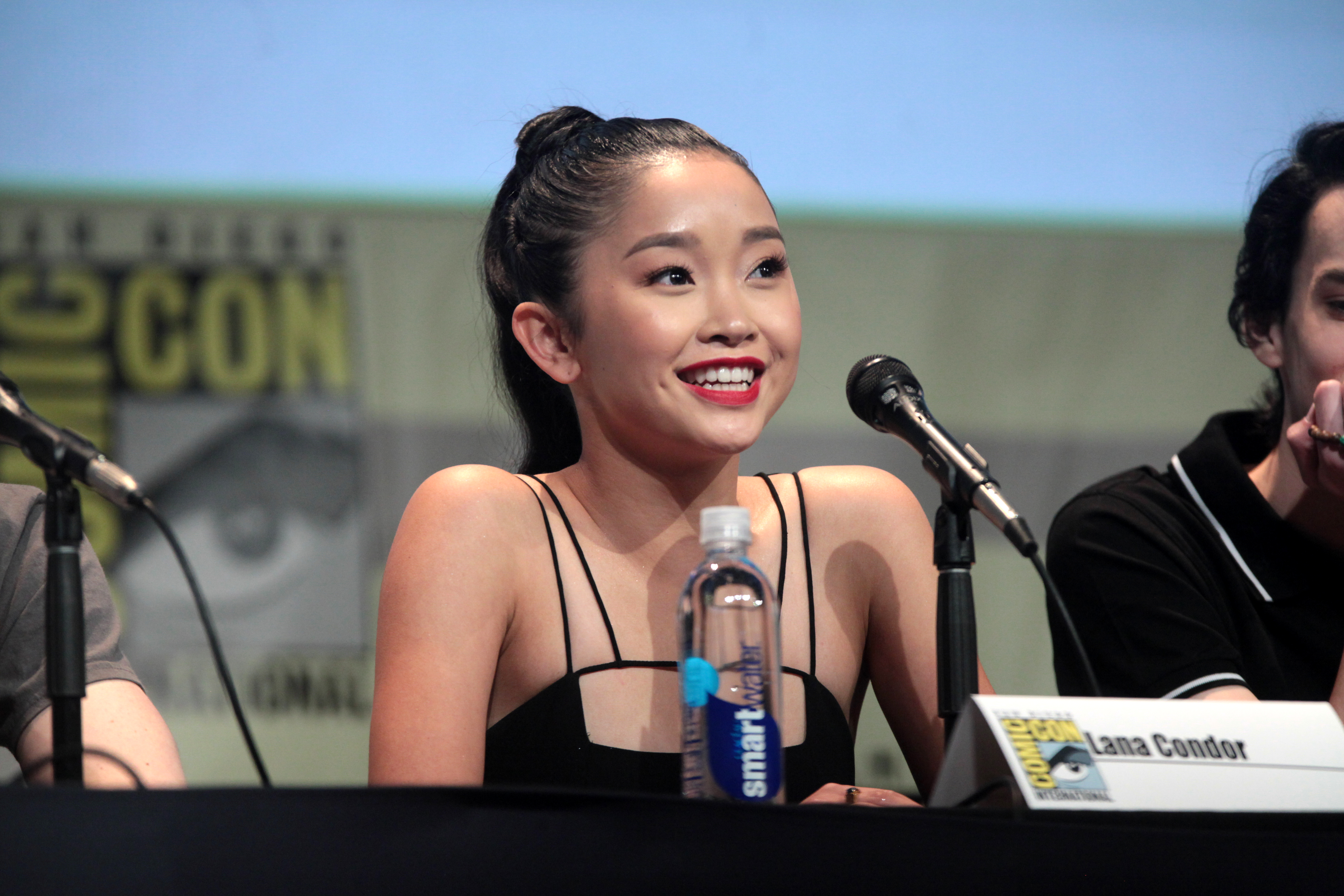This high-quality color photograph captures a young Asian woman with long dark hair, tied back, seated at a table at a Comic-Con event. She is wearing a strapless black dress and bright red lipstick, smiling and looking to her right. In front of her is a silver and black microphone, and a bottle of SmartWater. A white nameplate reading "Lana Condor" in black letters sits on the table, alongside a logo to the left in yellow, black, and blue with an eye that says Comic-Con. The black table she is sitting at is flanked by two people, one in a gray t-shirt on her left and the other in a black and white polo shirt on her right. The Comic-Con logo is visible in the blurred blue background, framing the scene with natural light and adding to the bright and clear setting. Lana Condor is the main focus, speaking into the microphone, reminiscent of a press conference atmosphere.